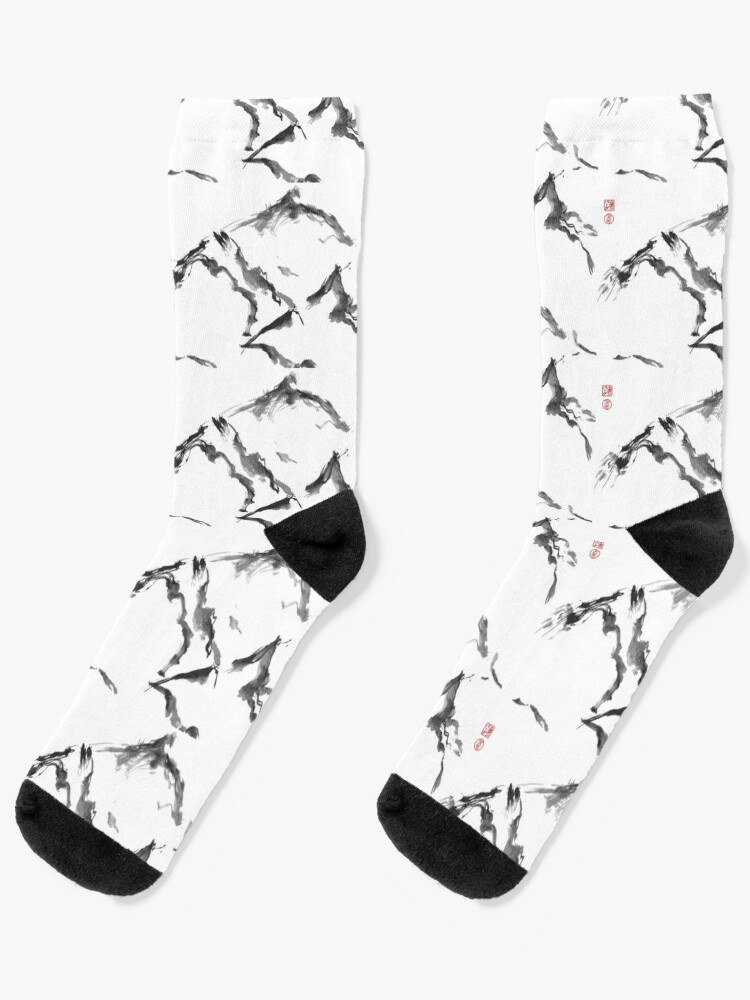This is a detailed color photograph of a pair of socks displayed against a plain white background. The socks are laid flat with the toes pointing toward the lower left hand corner and the heels toward the right. The socks feature solid black toes and solid black heel patches, likely for added durability. The main body of the socks is white with a black and gray marbled or watercolor-like pattern, resembling the look of a slab of marble. The sock on the right side has four evenly spaced small markings consisting of a circle and a square with something indistinct inside them, possibly a watermark or branding, which are not present on the left sock. The red markings that some described as potential characters are minimal and difficult to read. The socks are mid-calf length and appear to be intended for an online purchase, though there are no identifying texts or labels in the image.